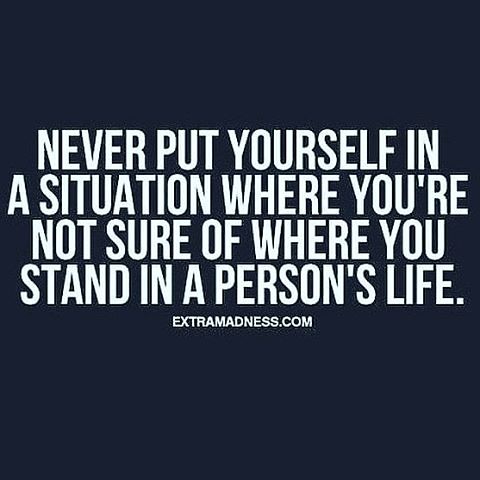This graphic design image features a typographic quote on a solid navy blue, square background. The quote is prominently displayed in bold, all-caps, condensed white sans-serif font, centered in the image. The text reads, "NEVER PUT YOURSELF IN A SITUATION WHERE YOU'RE NOT SURE WHERE YOU STAND IN A PERSON'S LIFE." Below the quote, in a smaller all-caps font, is the URL "EXTRAMADNESS.COM." The clean design focuses solely on the impactful quote, with the text occupying most of the space, slightly above the center of the image, creating a visually compelling and easy-to-read message.